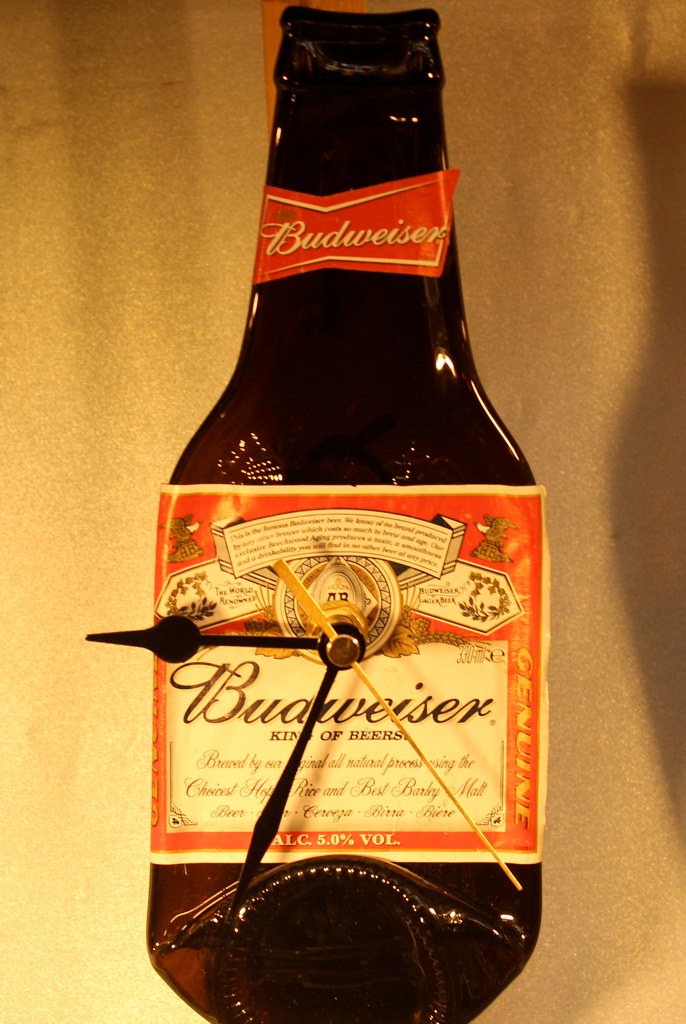This image captures a unique and intriguing clock that has been crafted from what appears to be an actual Budweiser bottle. The bottle has been expertly flattened without breaking, creating an interesting and distinctive shape. The bottom of the bottle extends slightly upward, adding to its eye-catching design. Prominently displayed on the bottle is the iconic Budweiser logo, featuring the classic red background with silver and white detailing, and proudly declaring Budweiser as the "King of Beers." The clock’s hour and minute hands are black, complementing the overall aesthetic, while a contrasting yellow second hand ticks around the face. Notably, the clock does not have numerical markers, requiring the user to estimate the time. This creative and functional piece seamlessly merges art with utility, making it a standout decorative item.